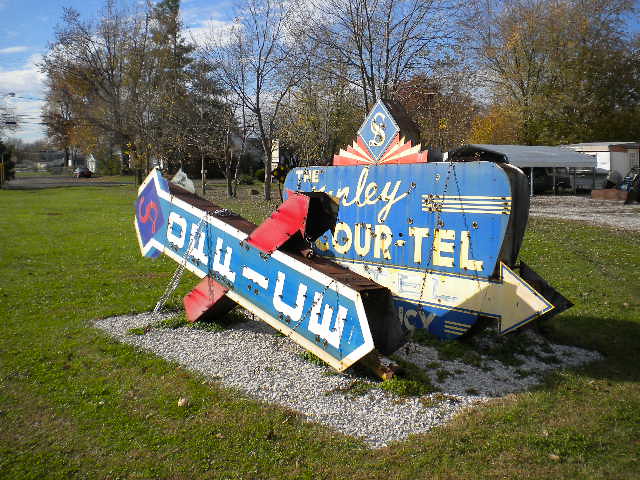This outdoor color photograph captures a close-up of a dilapidated motel sign propped on a pebbled square amidst a grassy lawn. The main sign, largely turquoise with rust and bullet holes, features cursive writing at the top, vaguely decipherable as "N-L-E-Y," followed by "O-U-R-T-E-L," and a large white arrow pointing to the right. The sign is topped by alternating red and white triangles, reminiscent of book pages, and a dark blue diamond containing an "S." In front of this stands a smaller sign, also in poor condition, reading "OFFICE" in white letters on a blue background, bisected by a red arrow, and marked by the same "S" in a diamond. Surrounding the signs, the grassy area transitions into a pebbled square, with light green grass dotted with trees exhibiting early autumn colors of yellow and red. The scene is further framed by a large white building to the left, a white shack with a light gray roof, a gazebo to the right, and sections of gravel. The sky above is bright blue with patches of fluffy white clouds, completing this nostalgic yet weathered landscape.